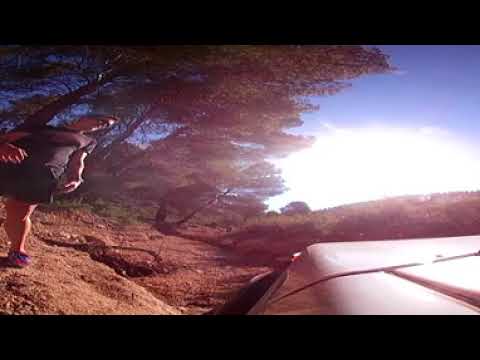The photograph captures an outdoor scene with a distinctive vintage quality, framed by thick black borders at the top and bottom, reminiscent of older camera styles. In the foreground, a man stands on a rocky, dirt-covered path that appears to be part of a hilly terrain. He is positioned on the left side of the image, donning a dark t-shirt, dark shorts, and bluish-purple sneakers. Sunglasses shield his eyes as he looks down, adding a casual, laid-back air to his stance.

Behind and to the right of the man, partially obscured by the angle, is a white vehicle—possibly an SUV or an upside-down boat—indicating some form of outdoor recreational activity like hiking or canoeing. The terrain around the vehicle is similarly rough and uneven, with patches of barren ground that might be interspersed with sparse, non-green grass.

The background is adorned with several tall, green-leaved trees, their brown trunks providing a stark contrast against the bright sky. Overhead, white clouds partially obscure the sun, which peeks through with an intense brightness, casting a glaring light across the scene. The overall composition is a bit unusual, giving the impression that the photograph was taken from a low angle, almost as if the photographer was lying on the ground.

This descriptive scene evokes an adventurous yet serene atmosphere, set against the backdrop of nature's raw beauty.